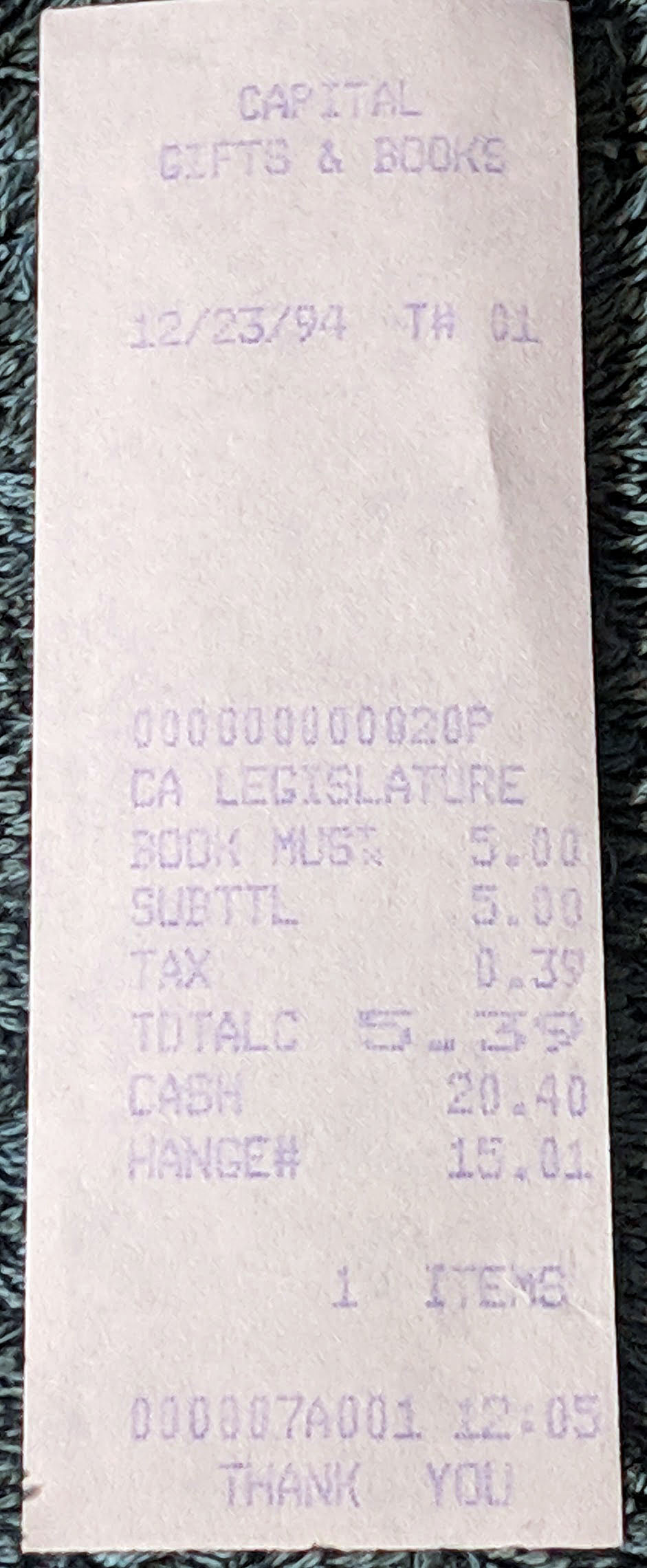A zoomed-in photograph of an old receipt from Capital Gifts and Books is shown on a dark, woven background, likely a black-and-blue or carpet-like material. The white receipt, slightly faded, features blue-purple text. The header reads "Capital Gifts and Books" with the date "12-23-94" just below it, indicating the purchase date. Following that, a code "TH-01-00000000020P" leads to the item purchased listed as "CA Legislature Book MUS" priced at $5. The receipt breaks down the costs with a subtotal of $5, tax of $0.39, resulting in a total of $5.39. The customer paid with $20.40 in cash and received $15.01 in change. A timestamp "000007A001-1205" indicates the transaction time at 12:05. Concluding the receipt, the message "Thank You" is printed at the bottom. The image is a detailed capture of a single-item purchase made decades ago, with the receipt occupying the majority of the frame.